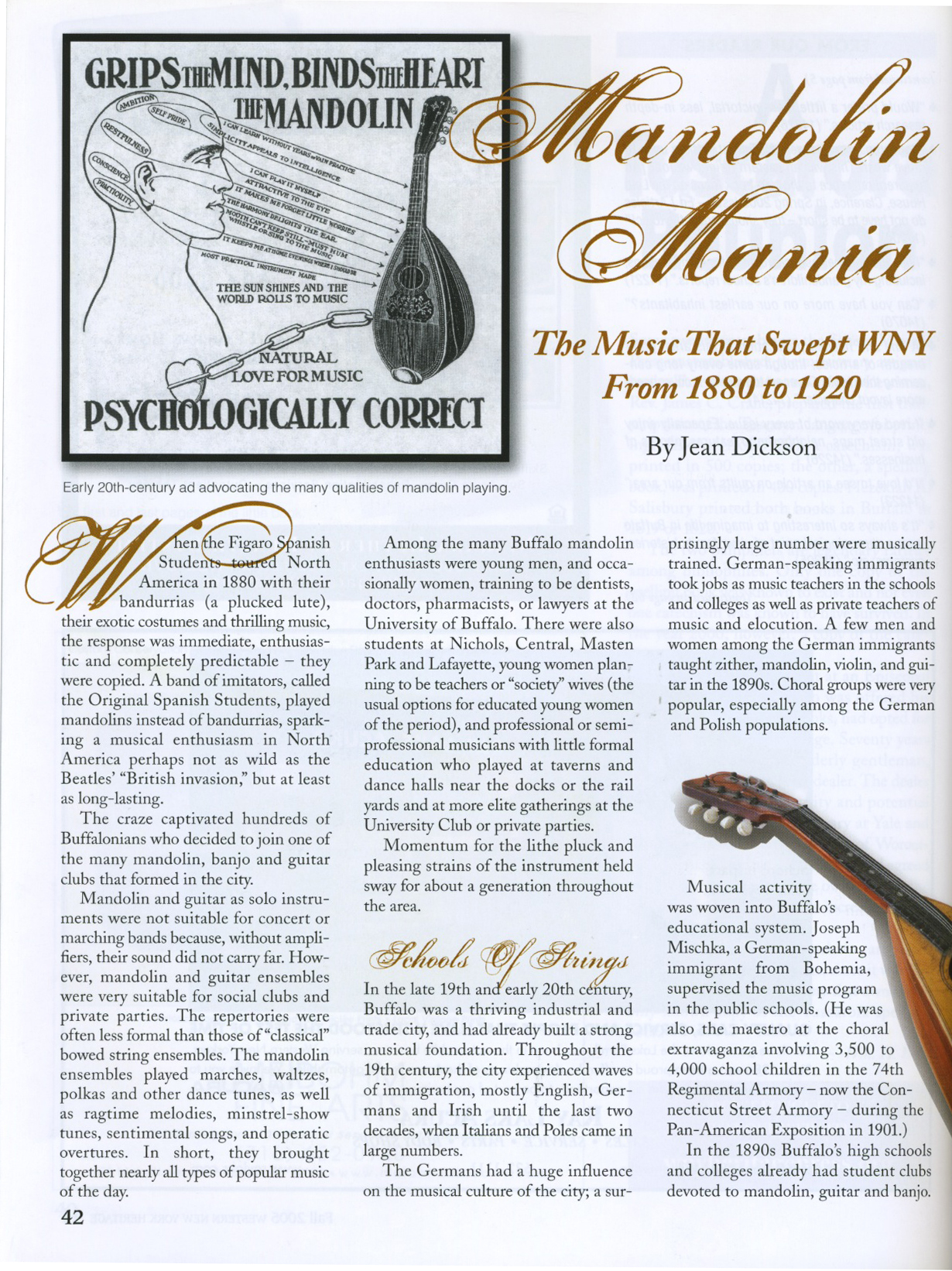This image is an intricately designed page from a music magazine that features an article titled "Mandolin Mania: The Music That Swept WNY from 1880 to 1920" by Gene Dixon. At the top right corner, the title is elegantly written in gold cursive. The left side of the page showcases a prominent square with a black border, containing an evocative graphic. This graphic includes a drawing of a person captivated by a mandolin, with a chain symbolically connecting the instrument to the person's heart and various arrows with words pointing towards the mandolin. Above this illustration, in bold font, it reads, "Grips the Mind, Binds the Heart, the Mandolin," and below the graphic, the phrase "Psychologically correct" is inscribed.

The main body of the article spans three columns on a white background. The first column begins with an ornate gold cursive "W" and halfway through, a gold cursive heading reads, "School of Strings." The article details the historical and cultural impact of the mandolin from the 1880s to the early 20th century in Western New York, mentioning the influence of Spanish students and their "bandurrias," the plucked string instruments they brought along with their distinct costumes and enthralling music.

Halfway down the third column, on the right side, there is an image of a mandolin. A similar heading "School of Strings" in gold cursive appears halfway down the column, tying the sections together. The depth of the article provides a rich exploration of the psychological and cultural significance of the mandolin through detailed textual and visual elements.